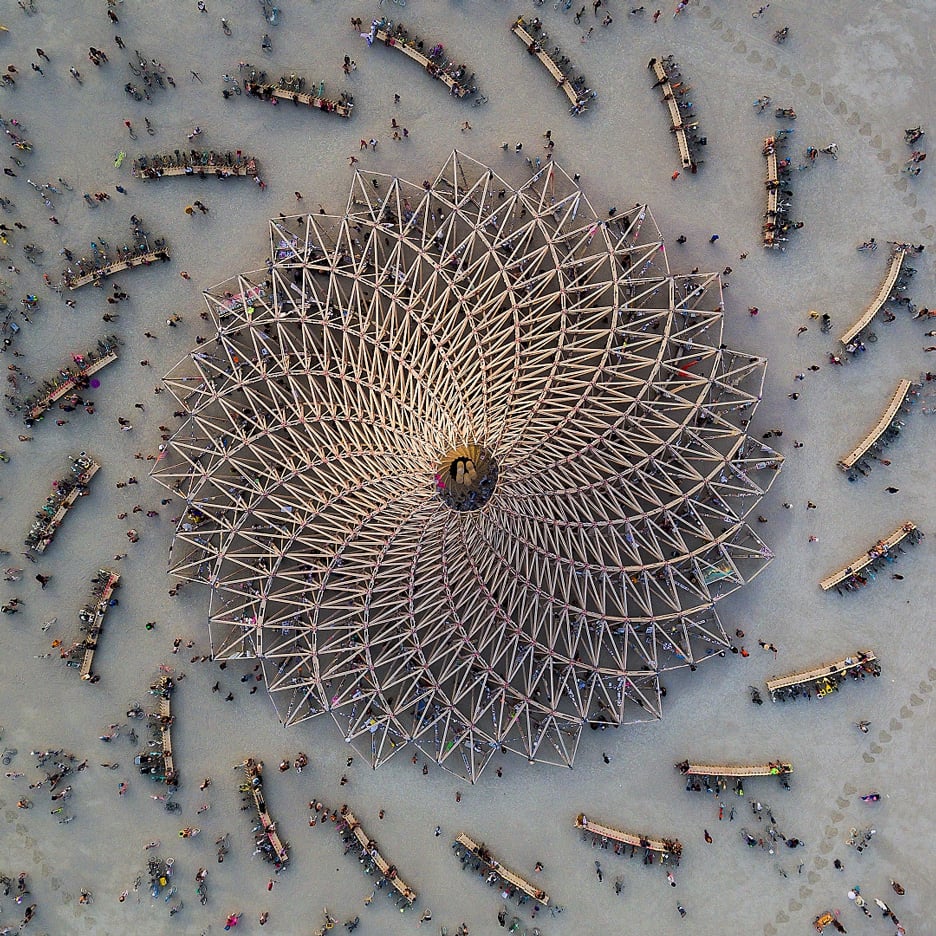The image is a bird's eye view of a giant spiral structure situated on a sandy beach. This swirly wooden construction, resembling a seashell or vortex, is at the center of the image and extends outward in a pattern strikingly similar to a mandala. At the top tip of the spiral structure, somewhat like a tent or hut with a painting or image adorning it, the spiral continues with zigzagging lines. Surrounding this central structure are numerous wooden benches and scattered people, emulating the spiral pattern. The people, appearing very small due to the overhead perspective, are wearing various colorful shirts, although the overall tone of the scene is neutral and beige. The beach is marked by footprints and other tracks, creating patterns in the sand along with the occasional wave visible in the top right corner, giving the impression of a lively festival or carnival-like atmosphere.